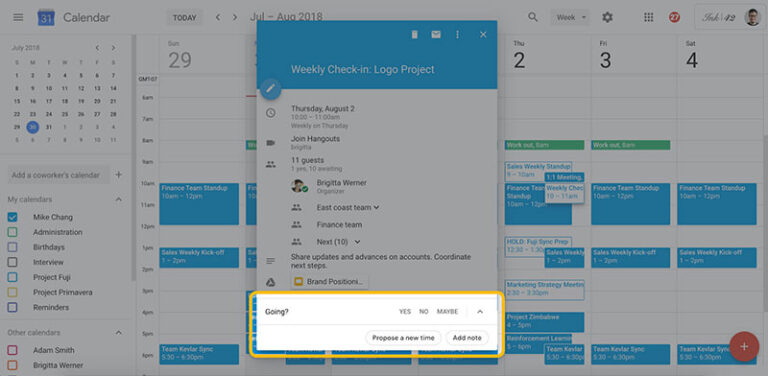The image depicts a screenshot of a Google Calendar account, likely associated with work. In the upper right corner, a small profile picture indicates that a user is logged in. Adjacent to the photo, the text "INC 42" appears in a cursive font, suggesting it could be the name of a business. Further to the left, a red circle displaying the number "27" in white text can be seen.

Centrally positioned on the screen is a dialog box for a calendar event titled "Weekly Check-In Logo Project," highlighted in white font against a light to medium blue toned background. The top section of this dialog box is distinctly marked by this blue background. Below the title, the event details are provided, stating that the meeting is scheduled for Thursday, August 2nd, from 10-11 a.m., and is set to recur weekly on Thursdays. It is mentioned that the meeting will take place via Hangouts, and Brigida Warner is noted as the organizer.

Towards the bottom of the dialog box, invitee response options are displayed, marked with "Going? Yes, No, Maybe." Additionally, there are options to propose a new time for the meeting or to add a note.